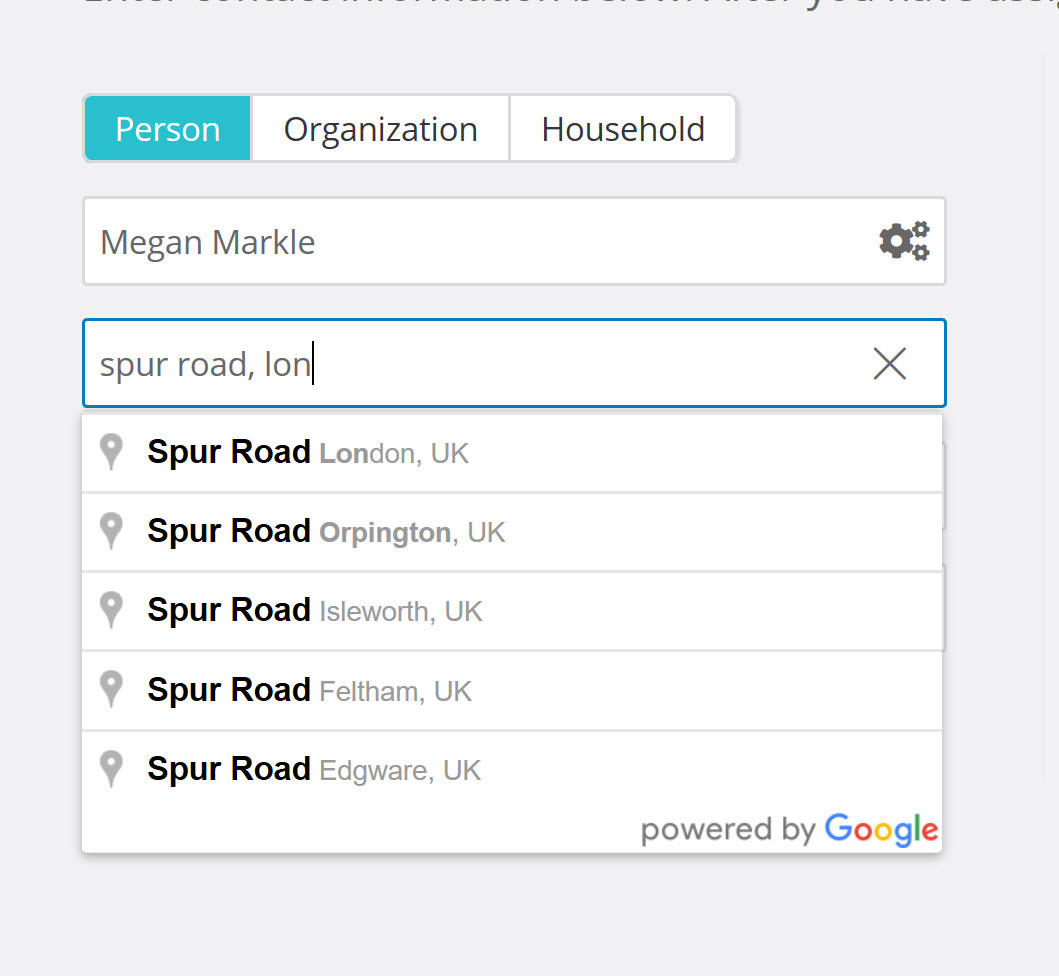The image features a light blue background with multiple user interface elements displayed prominently. At the top of the image, there are three distinct boxes: a blue one labeled "Person," and two white ones labeled "Organization" and "Household." Below these options, there is a large search bar where the user has typed "Megan Markle."

Underneath the search bar, there is a white box bordered in blue with a black 'X' icon on the right edge; the box contains the text "Spur Road, I own." Following this, five listings for "Spur Road" are displayed, each marked with a small gray pin that has a white circle in its center. The listings include:

1. Spur Road, London, UK
2. Spur Road, Orpington, UK
3. Spur Road, Islesworth, UK
4. Spur Road, Feltham, UK
5. Spur Road, Edgeware, UK

At the bottom of the image, the words "Powered by Google" are displayed, with the "Google" logo in its classic blue, red, yellow, and green colors. All these elements are enclosed within a large blue box that frames the entire content of the image.